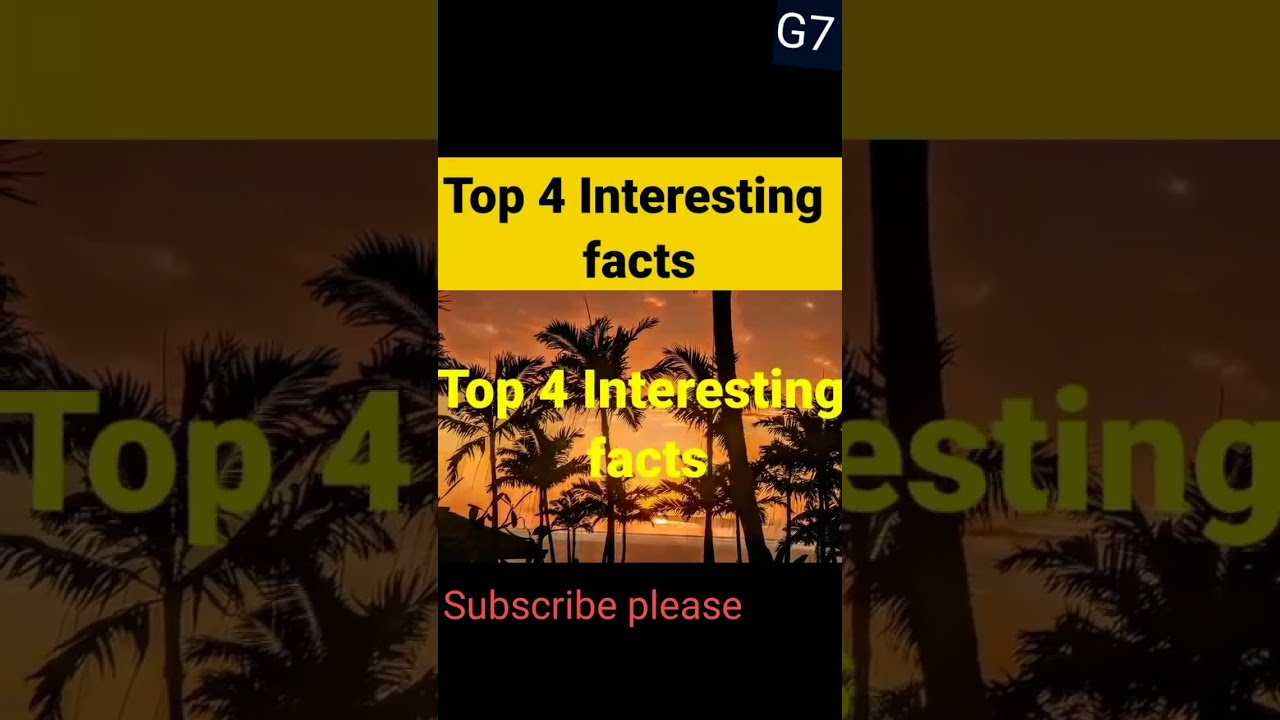The image is a promotional graphic in a vertical, portrait-oriented format, divided into three panels with the central panel being the focal point. The main central panel features a tropical-themed image framed by black margins at the top and bottom. At the very top, on a black background, in white text, it reads "G7" in the upper right corner. Directly below this, spanning the width of the panel, is a yellow rectangle with black text that reads "Top 4 Interesting Facts." Below this yellow banner is a scenic photograph of a tropical paradise, characterized by silhouettes of palm trees and possibly a hut, illuminated by the reddish-orange hues of either a sunrise or sunset. The distant horizon suggests either a body of water or low hills under the glowing sky. At the bottom of this central panel, on a black background, the red italic sans serif text urges viewers to "Subscribe please," with the "S" in "Subscribe" capitalized.

Flanking each side of this central panel are two other vertical panels that display zoomed-in, blurred, and blackened versions of the central image. These side panels subtly repeat parts of the "Top 4 Interesting Facts" text, with "Top 4" visible on one side and "Esting" discernible on the other, maintaining the tropical theme in a muted, out-of-focus manner.